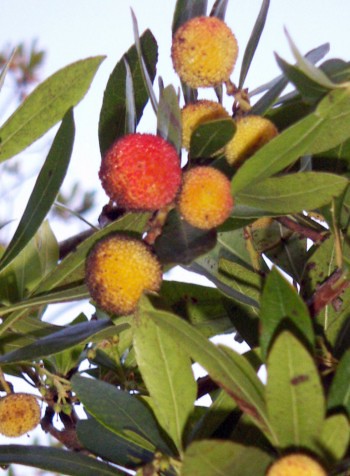The slightly out-of-focus photograph captures the unique strawberry tree, showcasing its distinctive, round, puffball-like fruits in various stages of ripeness, ranging from vibrant red to amber and green. Amidst the green, oval leaves, the image prominently features one central red fruit with six other fruits in close proximity, predominantly yellow and orange, arranged around it—three above and two below. The background reveals a hazy, bright day, accentuated by a flash that highlights the foreground elements. The overall scene is framed by the tree's foliage against a muted, bluish-gray sky, providing a serene and subtly colorful composition.